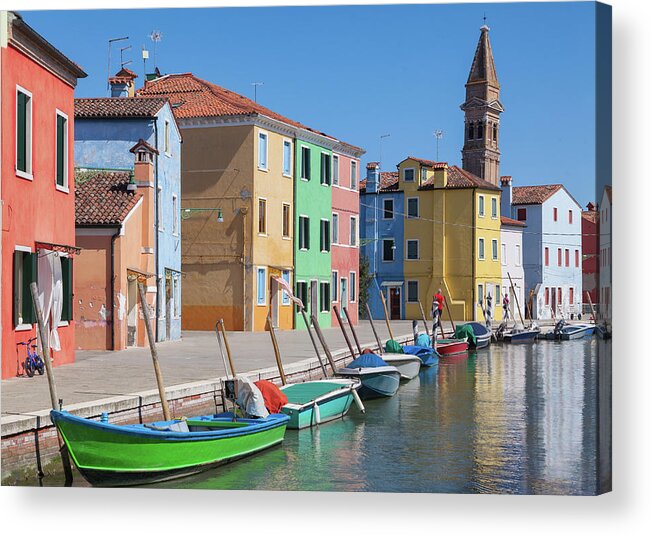This image, presented as a three-dimensional canvas print, captures a vibrant canal scene, likely in Venice, on a sunny day. The canal, filled with around ten colorful boats, cuts through the lower left corner of the photograph and gently curves toward the mid right. Each boat, including a prominent bright green vessel with blue trim at the front, features long wooden poles leaning against the gray, slightly curved sidewalk that runs parallel to the water. 

Lining the canal are nine multicolored buildings, ranging from red, brown, pink, and light blue to a unique structure split between yellow and blue. These buildings, mostly two to three stories high, showcase an array of bright pastels with matching rooftops, predominantly brown with visible chimneys. In the background stands a tall, brown brick spire topped with a cross, adding a historical touch to the scene. The sky overhead is a clear, vivid blue, reflecting the perfect weather. 

Despite the dynamic setting, the area seems quiet, with only a few distant figures visible on the sidewalk. The canal water mirrors the colorful facades, enhancing the picturesque charm of this quintessentially Venetian vista.